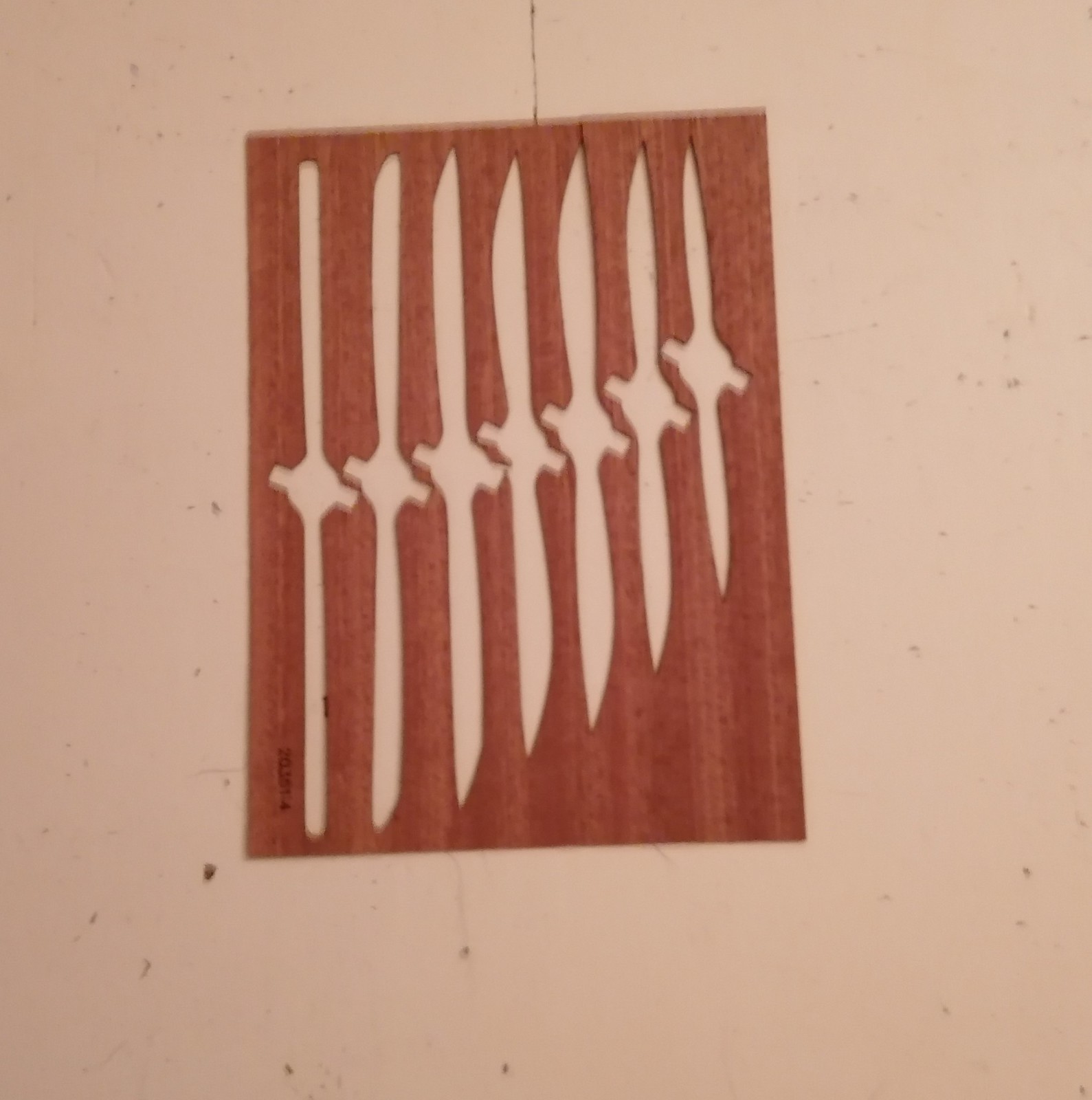This is a rectangular photograph slightly taller than it is wide, showcasing a reddish-brown stencil-like wooden piece placed against a creamy rose-colored, somewhat dingy background with black marks and specks. The wood appears flimsy and weathered, featuring a series of seven distinct cutouts arrayed from tallest to shortest, resembling either propellers or knives. Each cutout consists of a round space in the center with elongated, variably shaped extensions: some straight, some curved, and others pointed, mimicking blades. The carving has varied rectangle lengths and shapes emerging from the top and bottom of these central circles. There's an almost hieroglyphic-like series of numbers or writing at the bottom left, difficult to decipher but possibly including the digits 2, 0, 3, 5, 1, and 4. Overall, the piece has the appearance of a carefully designed template, possibly used for etching or as an artistic representation.